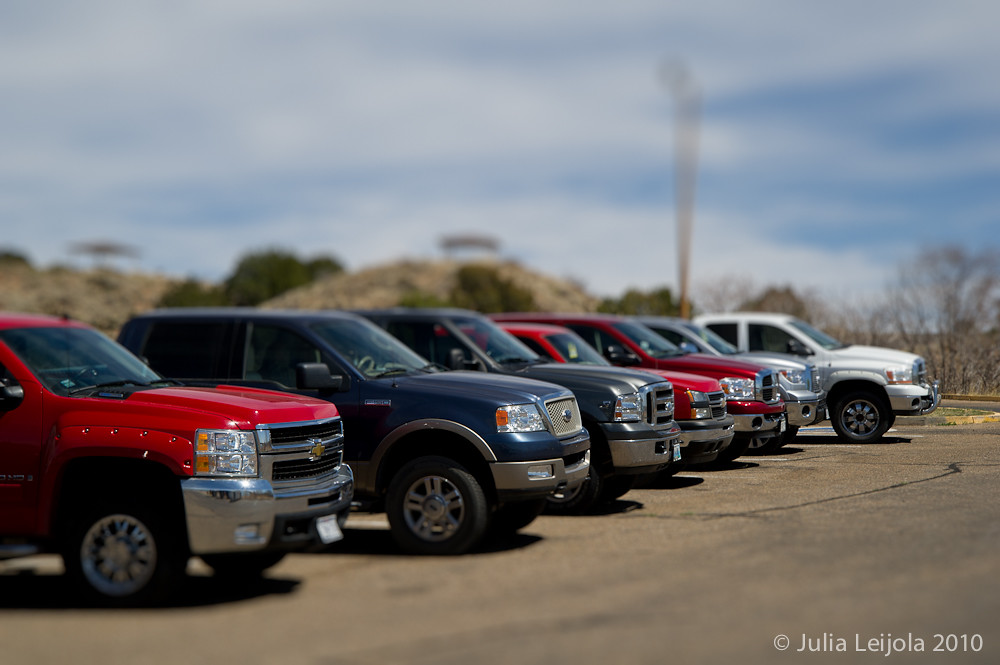The photograph, captured by Julia Lejola in 2010, depicts a parking lot under a sky of vibrant blue with light gray clouds. In the blurry background, a picturesque row of trees intermingles with a hilly landscape. Some trees boast lush green leaves while others stand bare. The asphalt surface of the parking lot appears faded and well-worn. Parked within the lot is a row of six or seven vehicles, predominantly van-shaped, featuring an array of colors including red, blue, silver, black, and white. Among these cars, which include makes such as Ford, Chevy, and Toyota, a silver car protrudes slightly forward from the lineup. Sunlight casts distinct shadows beneath the vehicles, emphasizing their varied colors and models. The image is marked with a copyright watermark in the bottom right corner that reads "Julia Lejola 2010."